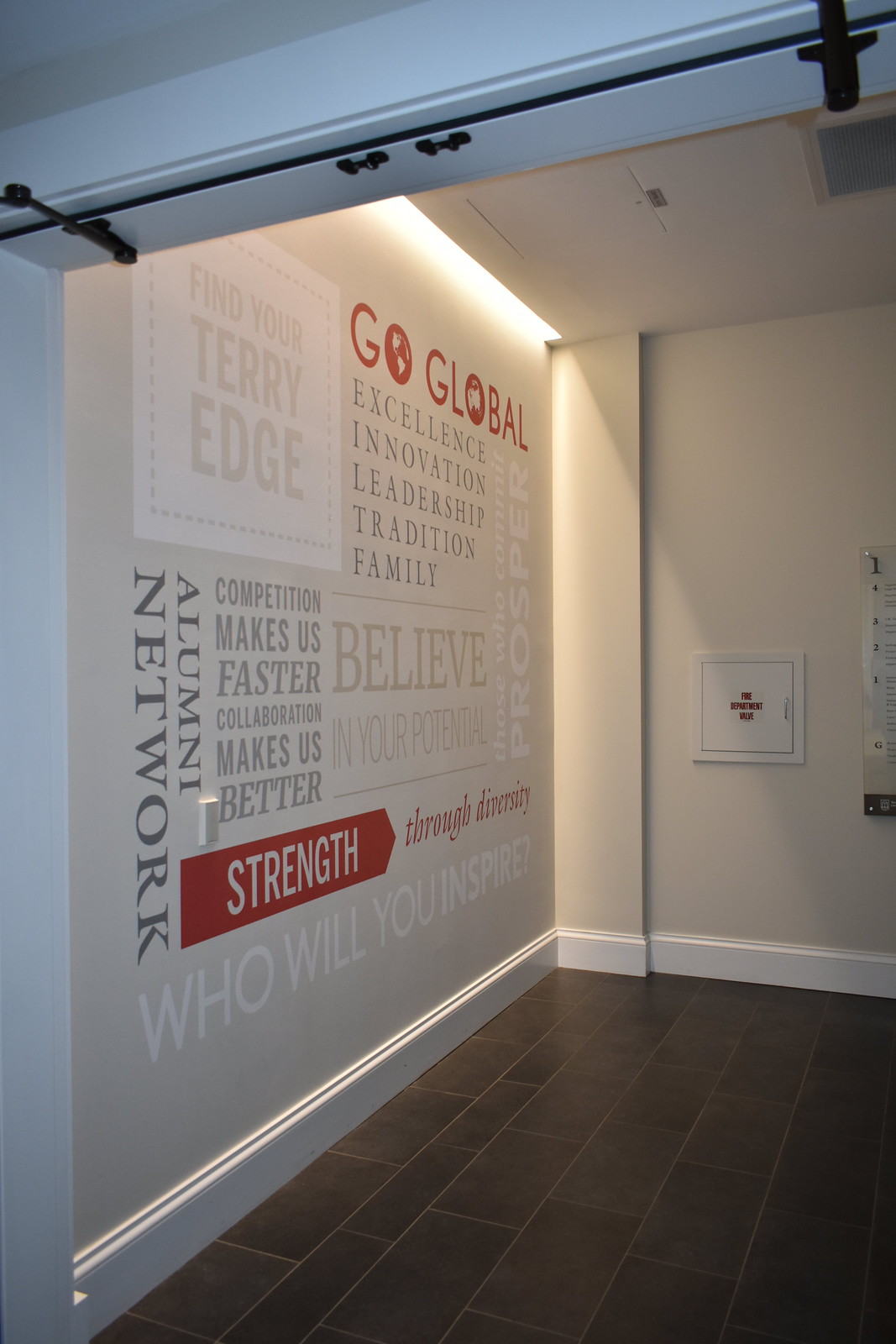This photograph captures the corner of a room within a building, featuring a dark or black tiled floor. The walls are primarily beige with white trim, and various inspirational messages are prominently displayed in red, black, and white text. The central theme is "Go Global," with words such as "Excellence," "Innovation," "Leadership," "Tradition," "Family," "Believe in Your Potential," "Strength," and "Who will you inspire?" prominently visible. Additional text includes "Find Your Terry Edge" and "Alumni Network." The upper portion of the wall, near the ceiling, is illuminated, highlighting these motivational messages. There is also a fire extinguisher and an emergency box attached to the opposite wall. The ceiling features an air conditioning vent.